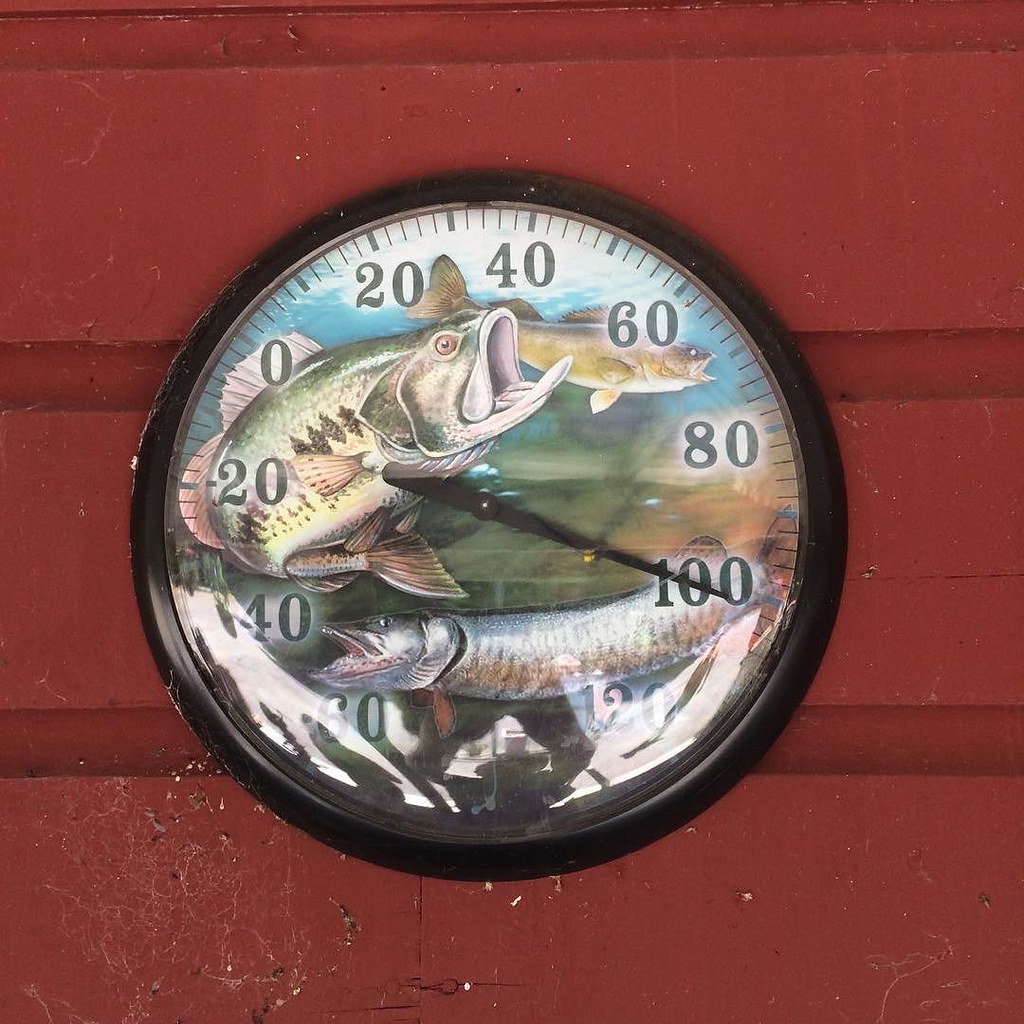This image captures a vintage outdoor thermometer, measuring temperatures from -60 to 120 degrees Fahrenheit. The thermometer's face is adorned with a charming illustration of three fish, including a bass with its mouth open and a pickerel, all swimming in a painterly depiction of water. True to its era, the outer edge of the thermometer is encased in a black metal ring, adding to its nostalgic character. The thermometer is mounted on a vibrant red painted wall that has collected a few spider webs, suggesting it's in an outdoor setting. Such thermometers, popular in the 1970s, are commonly found in antique shops and are often seen at campgrounds, fitting perfectly with their rustic ambiance. On this sunny day, the thermometer reads a sweltering 100 degrees Fahrenheit, indicating a hot summer afternoon.